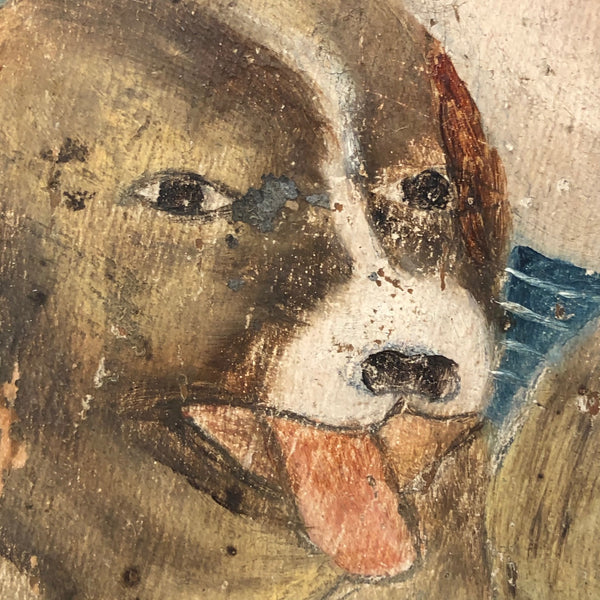This vibrant and detailed painting captures the joyful expression of a brown and white dog with an open mouth, panting happily. The dog's expressive brown eyes gleam with cheerfulness. His tongue is out, and no teeth are visible, enhancing his friendly demeanor. His head is adorned with long, fluffy brown ears, and the white patches are noticeable in the middle of his face, between his eyes, and around his nose. The background is a blend of pale brown, blue, and white, adding a serene touch to the image. The painting is well-illuminated with natural light, highlighting the clear and bright setting. Though parts of the painting appear slightly chipped, the overall image quality remains high and free from distractions such as people, other animals, or text.